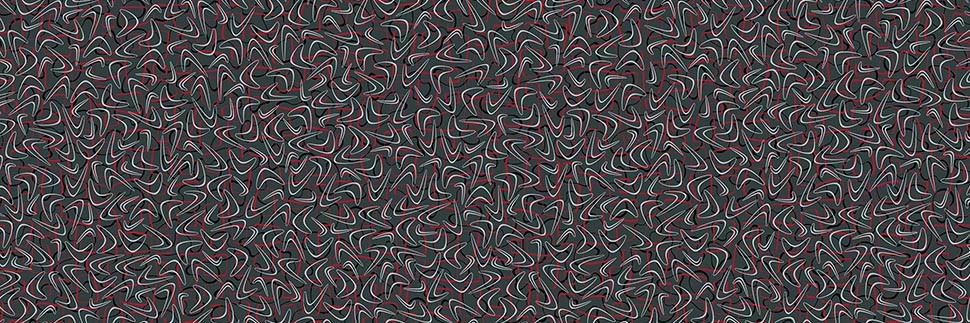The image displays an abstract pattern featuring a dark gray background densely covered with small, white-outlined boomerang shapes. Scattered amongst the white boomerangs are black-outlined boomerang shapes, adding another layer to the intricate design. Additionally, there are sporadic, red, rounded rectangles and black, bowtie-like shapes, all contributing to the complex, jumbled arrangement. The pattern is evenly distributed with no single element dominating the composition. The image is significantly wider than it is tall, approximately four times as wide, creating a sense of expansive repetition. The overall effect is reminiscent of an optical illusion, inviting viewers to discern hidden messages or shapes within the abstraction.